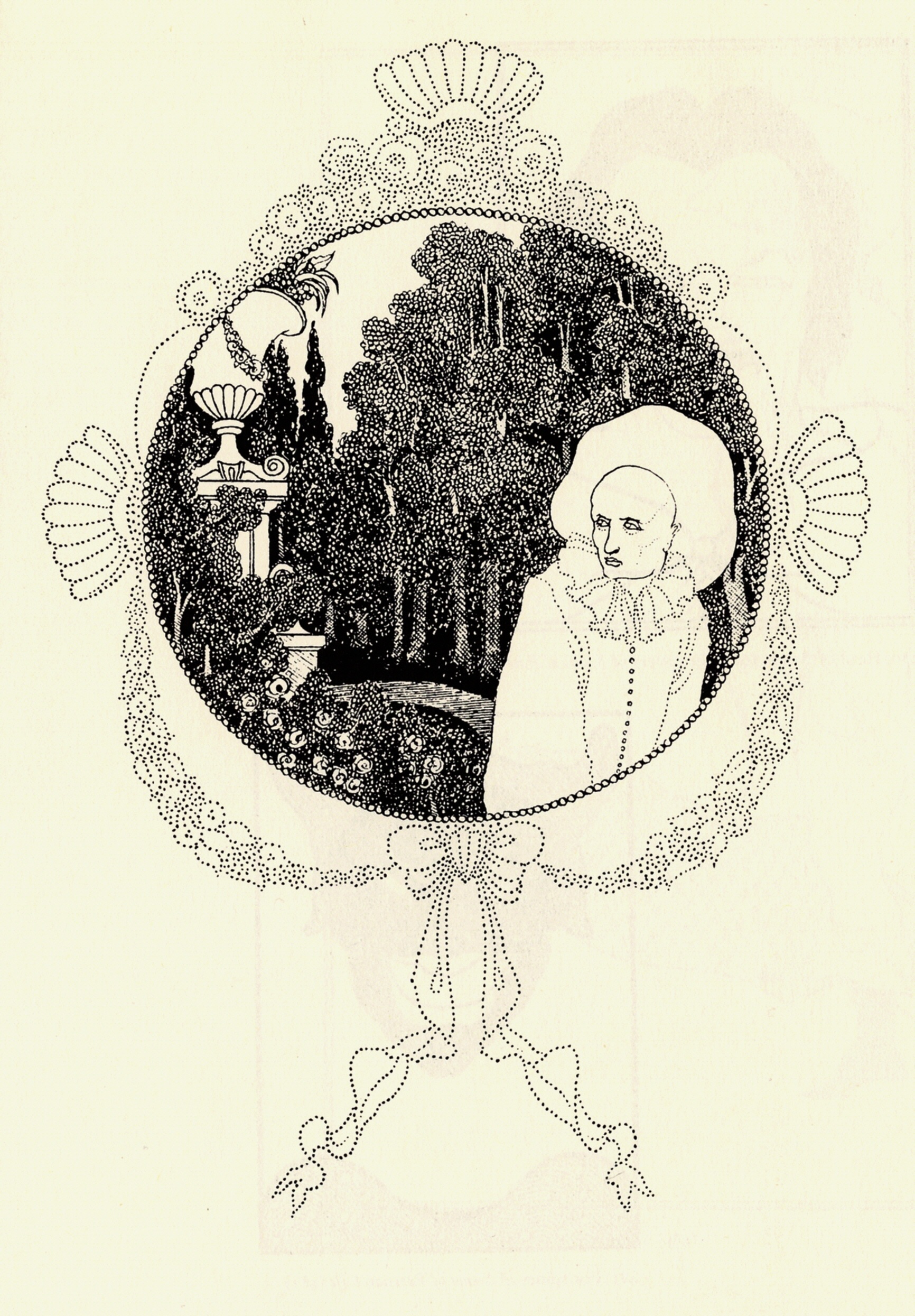This intricate black and white artwork, possibly created using lithography or a fine-point pen technique, is set on a rectangular, cream-colored background. At the centerpiece is a large, circular frame adorned with decorative embossing of seashells and floral motifs at the top, left, and right, with a ribbon bow hanging below. The scene within this circular frame depicts a lush garden filled with numerous tall trees, abundant flowers, and a stone walking path. Amidst this natural setting, there stands a bald figure dressed in Renaissance-era clothing, featuring a large white flounced collar and a long-sleeved robe with many buttons down the front. Positioned in the garden background is an elaborate 16th-century-style statue holding a large cup, anchoring the historical ambiance of the piece.